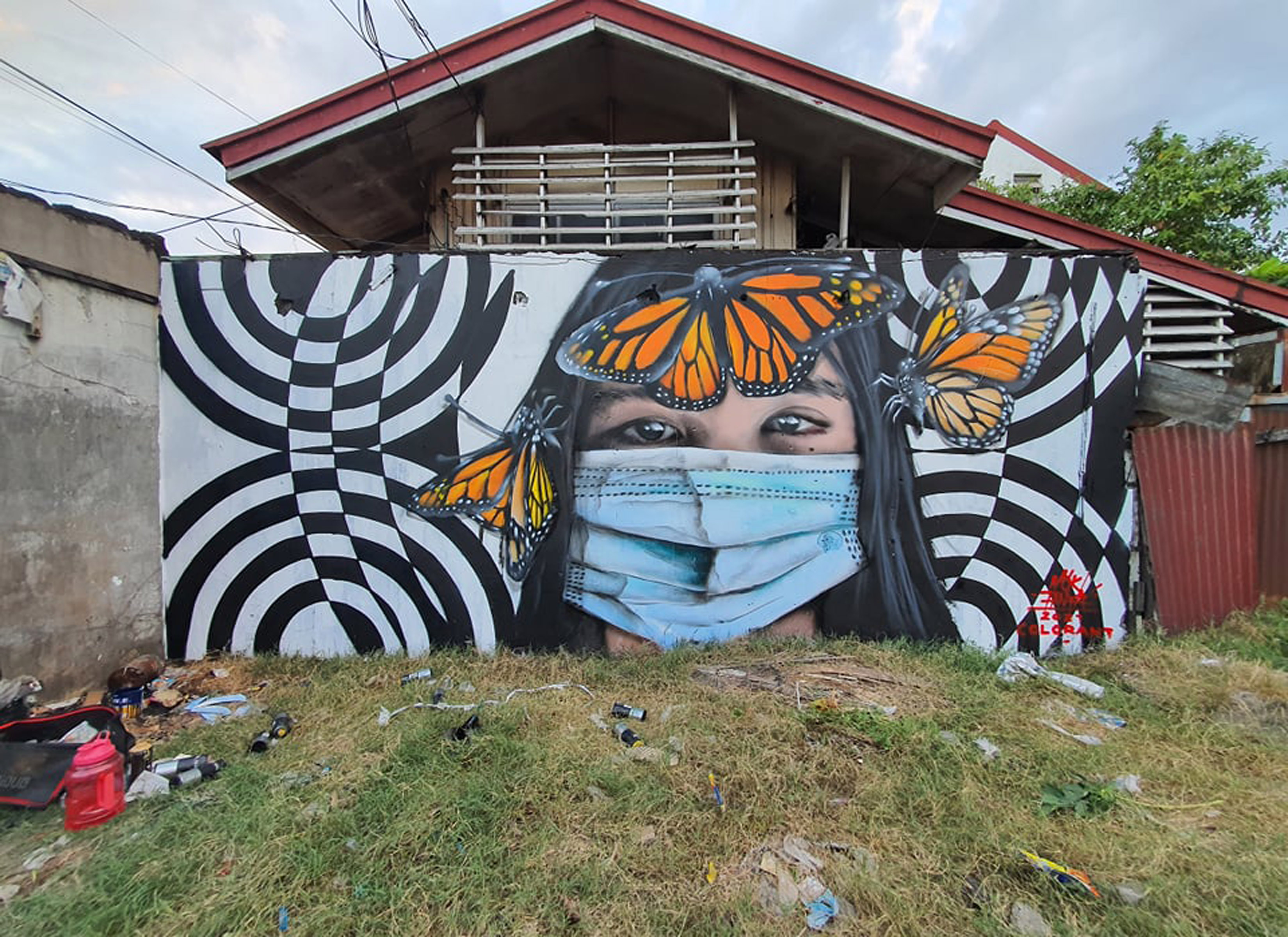The image features a striking mural painted onto a wall within an empty lot, surrounded by an unkempt patch of grass strewn with garbage, including distinguishable red water jugs and broken beer bottles. The mural is dominated by intricate black and white intercut spirals forming a complicated pattern. At its center is the realistically rendered face of a young woman with long, dark, straight hair, wearing a blue surgical mask. Three oversized monarch butterflies, each the size of half her face, perch delicately, one on her forehead and one on each side of her head. The mural has a small red signature in its lower right corner. To the left of the mural stands a concrete wall, while to the right is a red piece of metal siding. Behind the mural, the top of a worn-down building with a red pitched roof and white under trim is visible. The house features a wooden porch fence in disrepair. In the background, the sky is overcast with clouds, and power lines hang in the upper left, while a tree’s branches appear just barely visible in the upper right.